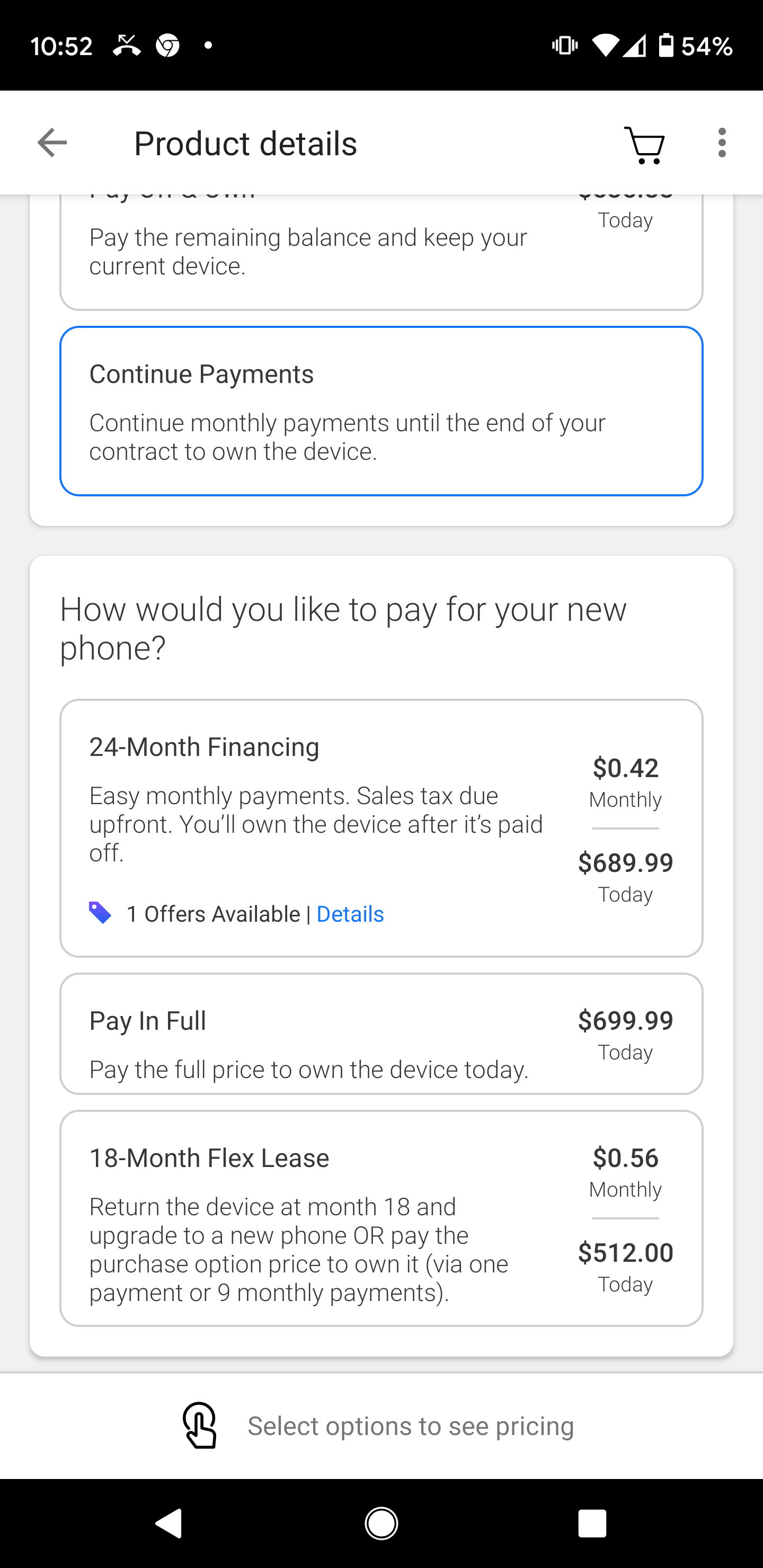The image is a screenshot captured on a mobile device at 10:52 AM, as indicated by the black bar at the top of the screen. On the right side of this bar, there is a missed call icon, and the battery level shows a 54% charge. Below this, a white bar spans the screen with the text "Product Details" on the left and a shopping cart icon on the right.

The background beneath is gray, and it encloses a white box that contains various options and buttons. The first button is labeled "Pay the remaining balance and keep your current device." Below this, a blue-outlined button says, "Continue monthly payments until the end of your contract to own the device."

Following these elements is the question, "How would you like to pay for your new phone?" with three payment options:

1. **24-month financing**: $42.42 per month, totaling $689.99. This option includes easy monthly payments with upfront sales tax. You'll own the device once it’s paid off.
2. **Pay in full**: A single payment of $699.99 to own the device immediately.
3. **18-month Flex lease**: Return the device at the end of 18 months to upgrade to a new phone, or pay the purchase option price to own it via one payment or nine monthly payments. This option costs $50.56 per month, with an upfront fee of $112.

At the bottom, the text instructs to "Select options to see pricing."